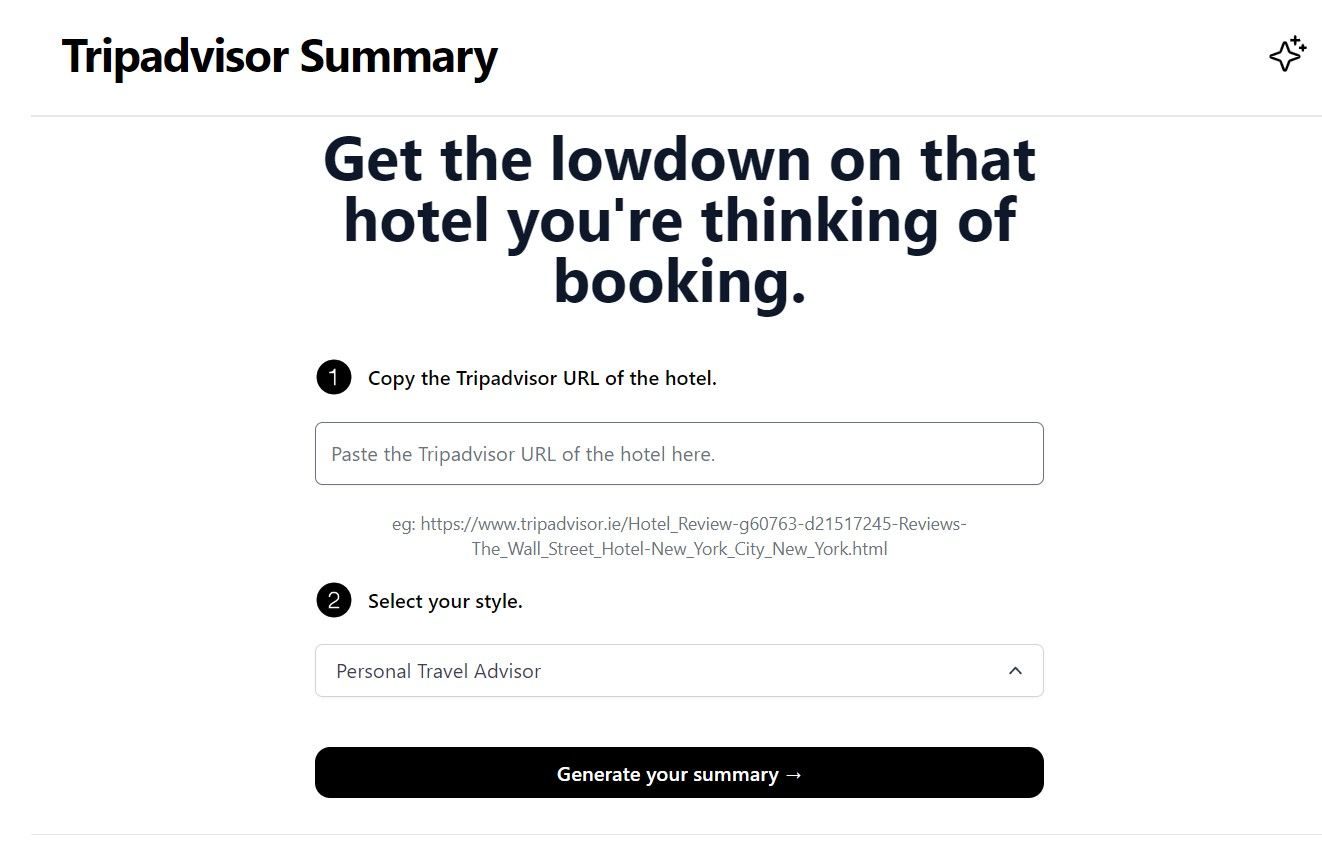**Caption:**

A detailed screenshot of a Trip Advisor Summary web page. The title "Trip Advisor Summary" is prominently displayed in bold, large black letters on the top left side of the header. The web page background is predominantly white, matching the header’s background.

In the middle of the screen, a message reads: "Get the lowdown on all the hotels you're thinking of booking." Below this, there are two main sections:

1. The first section, marked with a black circle containing the number "1," instructs users to "Copy the Trip Advisor URL of the hotel." Below this instruction is a search bar, accompanied by an example URL format (e.g., tripadvisor.ie/hotel_review).

2. The second section, indicated by a black circle with the number "2," prompts users to "Select your style" from a drop-down menu. The first available option in this menu is "Personal travel advisor."

At the bottom of the second section is a prominent black button labeled "Generate your summary."

Additionally, a four-pointed star outline is visible in the top right corner of the header. The overall design is minimalistic, drawing attention to the functional elements of the page.